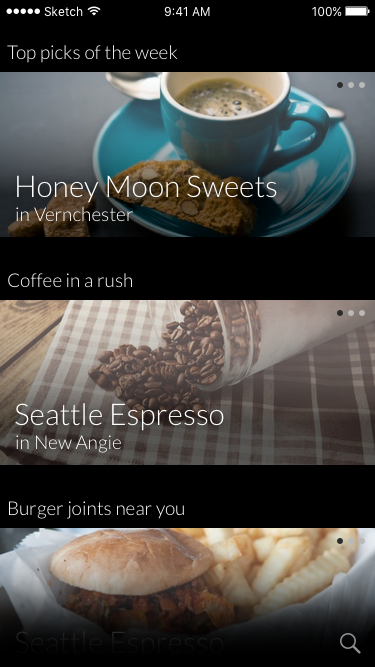This screenshot, captured from a phone, showcases various elements with meticulous detail. In the top-left corner, the phone displays full signal bars and the time, 9:40. On the right-hand side, a battery icon indicates a full charge at 100%. The background of the screenshot is black, making the visuals stand out.

The content is divided into three main sections, each highlighting something different. 

1. **Top Pics of the Week**: This section features a visually appealing image of a small blue plate with a matching blue coffee mug containing black espresso. A spoon rests behind the mug. Accompanying the coffee is a piece of bread, possibly a scone with nuts, all set on a black table. The caption reads "Honeymoon Sweets in Vernchester" and mentions the theme "coffee in a rush."

2. **Seattle Espresso in New Angie**: Below the first section, this part features a rustic display of coffee beans being poured from a glass jar onto a brown and white checkered cloth spread over a wooden table. This setup emphasizes the artisanal nature of the coffee experience.

3. **Burger Joints Near You**: The final section showcases a delicious burger and fries ensemble. The crinkle-cut fries and the white-waxed paper beneath the meal add to the presentation. The burger seems substantial, possibly a pulled pork style, with a soft white bun. In the bottom-right corner, there is a magnifying glass icon, suggesting the possibility of exploring more options, but the screenshot cuts off at this point.

Overall, the screenshot serves as a detailed, visually engaging display of curated food and beverage options.